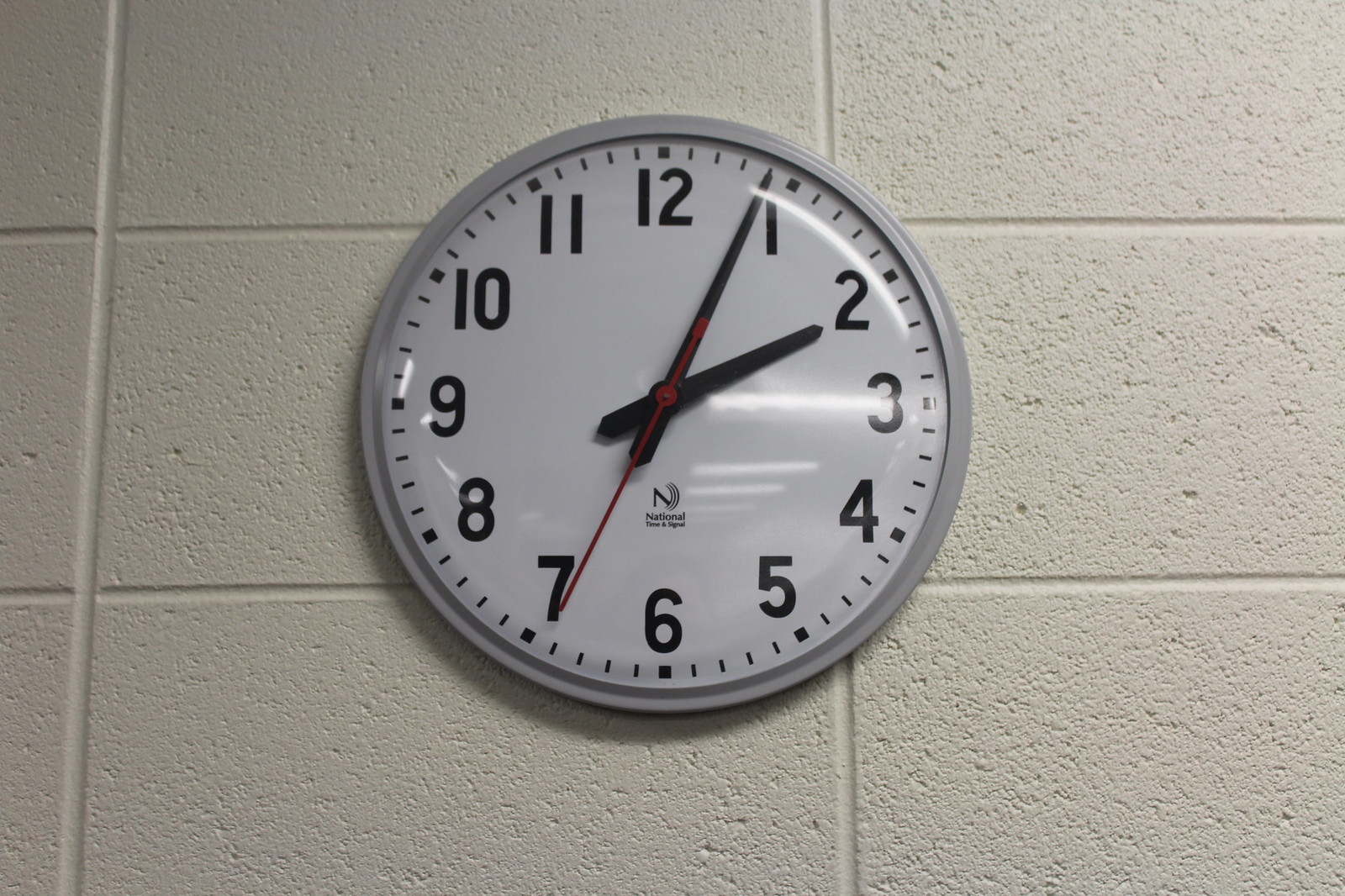This color photograph depicts a circular wall clock mounted on a neatly painted white cinder block wall. The wall comprises large, uniformly painted cinder blocks, including the grout lines, giving it a clean and well-maintained appearance. The clock, enclosed in a light gray or silver plastic frame, features a white face with black numerals and minute markers in the form of small dashes between the numbers. The clock hands are black, with the hour hand pointing at 2 and the minute hand slightly past 1, indicating the time as 2:04. The second hand, the only element in vivid color, is red and positioned at the 7. A glass or plastic cover protects the clock face, reflecting rows of fluorescent ceiling lights, creating noticeable glare lines on the surface. Below the clock's hands, the word "National" is faintly visible.